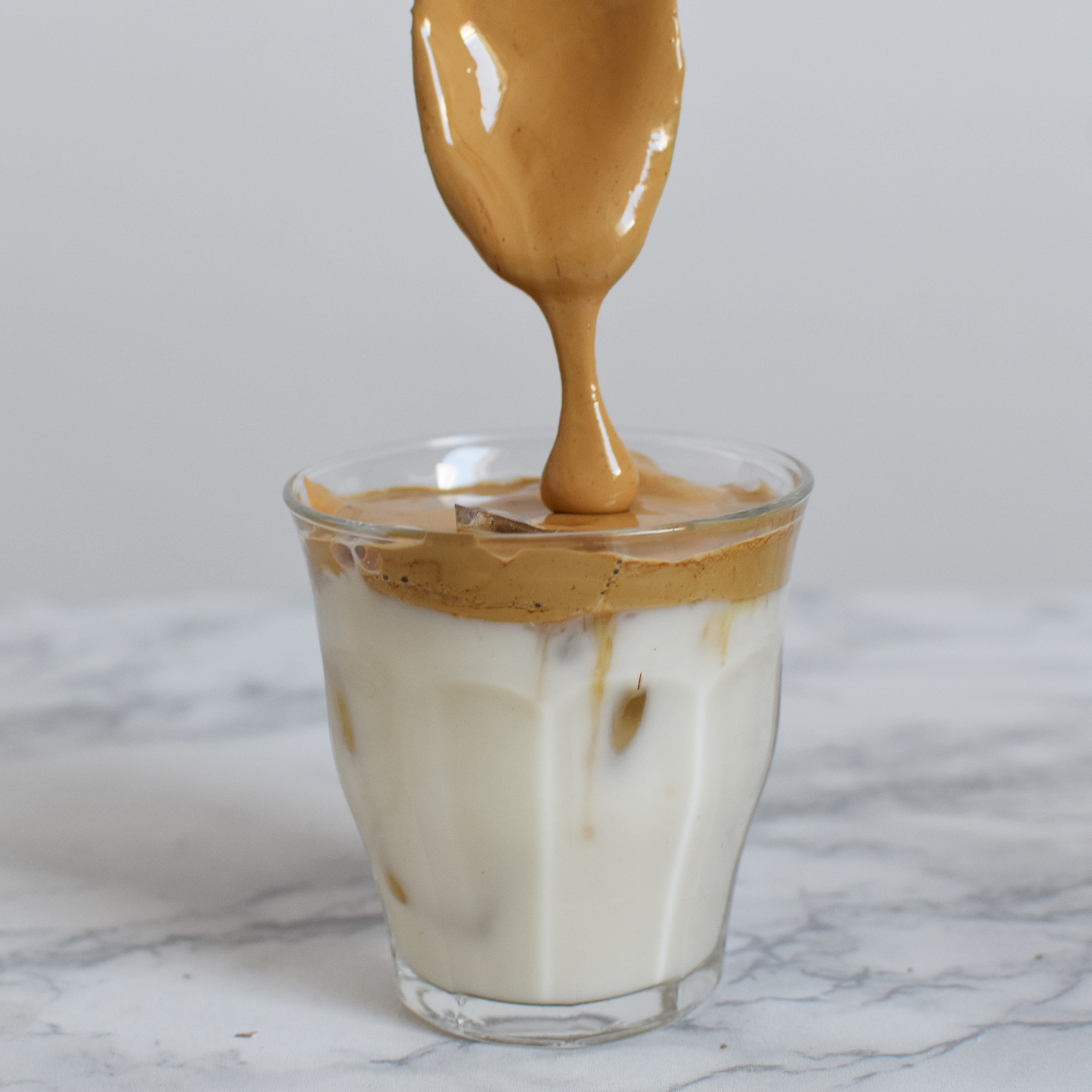This photograph features a clear, short, and slightly faceted glass sitting on a marble counter with a white and gray marble pattern. The glass contains a creamy white substance that resembles ice cream or frozen yogurt, potentially flavored with coconut or butter pecan. Atop the ice cream is a rich, gooey brown topping that looks like caramel or chocolate. A spoon held above the glass is dripping this gooey caramel or chocolate sauce onto the dessert. There are no ice cubes visible in the glass, but there is a bulk piece of chocolate floating on top. The scene is set on a clean marble surface with no people present in the photo, focusing entirely on the delectable dessert.